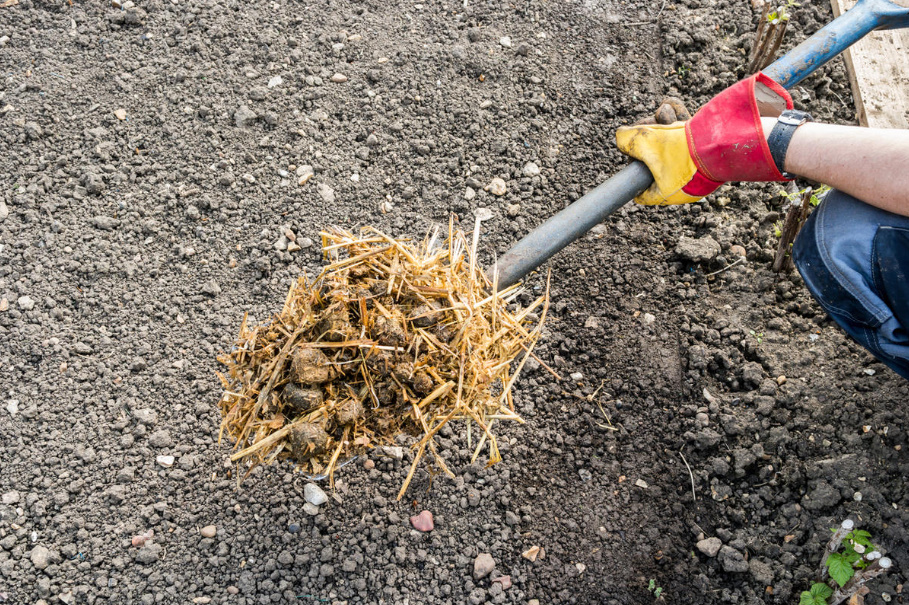In this rectangular image, a worker is seen scooping something off the ground with a shovel. Only the worker's knee and arm are visible. He is wearing jeans, a wristwatch with a black wristband, and yellow and red rubber gloves. The shovel he is using has a worn-out blue handle and a black base. The contents he's scooping appear to be straw mixed with what looks like animal droppings, similar to mucking out a horse stable. The ground in the background is a mixture of bare dirt with small rocks and some leaves, and a green plant is visible in the bottom right corner. Additionally, a wooden plank is barely visible in the top right corner, hinting it could be part of a larger structure just out of the frame.